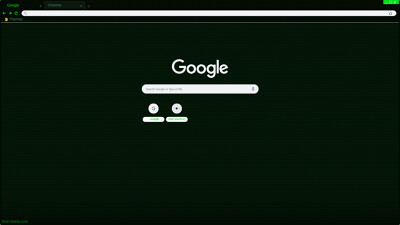The image is a small, horizontally-oriented screen capture of a computer screen, measuring approximately two inches high and three inches across. The background of the image is entirely black. At the top, there is a blank white address bar stretching from the left to the right. Above the address bar, lime green text is visible, potentially indicating a browser UI element. In the upper right corner, a green bar is faintly discernible. Below the address bar, in the middle of the screen, the word "Google" is displayed in white letters, followed by an elongated, rounded rectangular search bar. Beneath this search bar, there are two white circles side by side, and underneath each circle, there are short, rounded rectangular white lines. The overall impression is of a reduced-in-size screenshot of the Google homepage. The details within the image are somewhat blurry, particularly around the chooser circles and their corresponding labels.